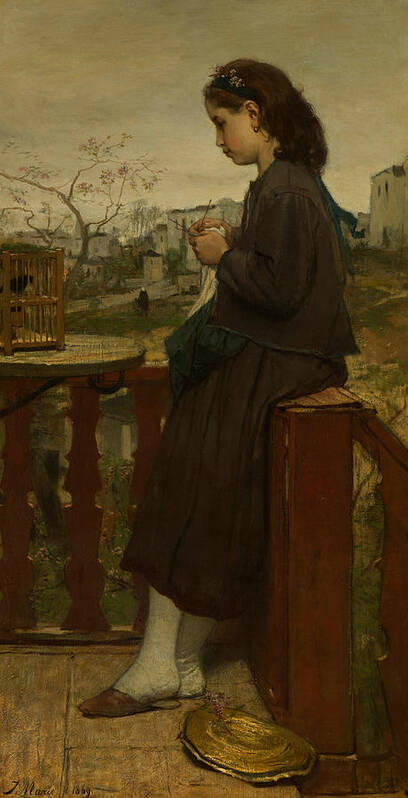The painting titled "Girl Knitting on a Balcony" by Jacob Maris depicts a young girl, approximately 12 or 13 years old, seated on the right-hand side of a wooden-railed balcony or porch. The artwork, likely created in the mid-19th to mid-20th century, showcases the girl leaning against a brown post of the balcony. She is dressed in a brown skirt and top with white tights and brown slippers. Her long hair reaches her shoulders and she is holding a knitting needle and black-and-white yarn, focusing intently on her knitting. At the bottom right corner rests a straw hat. To her left, a round table holds a birdcage with a bird inside, positioned on the flat part of the banister. The background reveals a misty, gray sky suggesting an impending storm, a sparse tree with few leaves, and a small village with white houses and reflective water. The overall style of the painting is realistic, capturing a serene and contemplative moment of the girl amidst her surroundings.